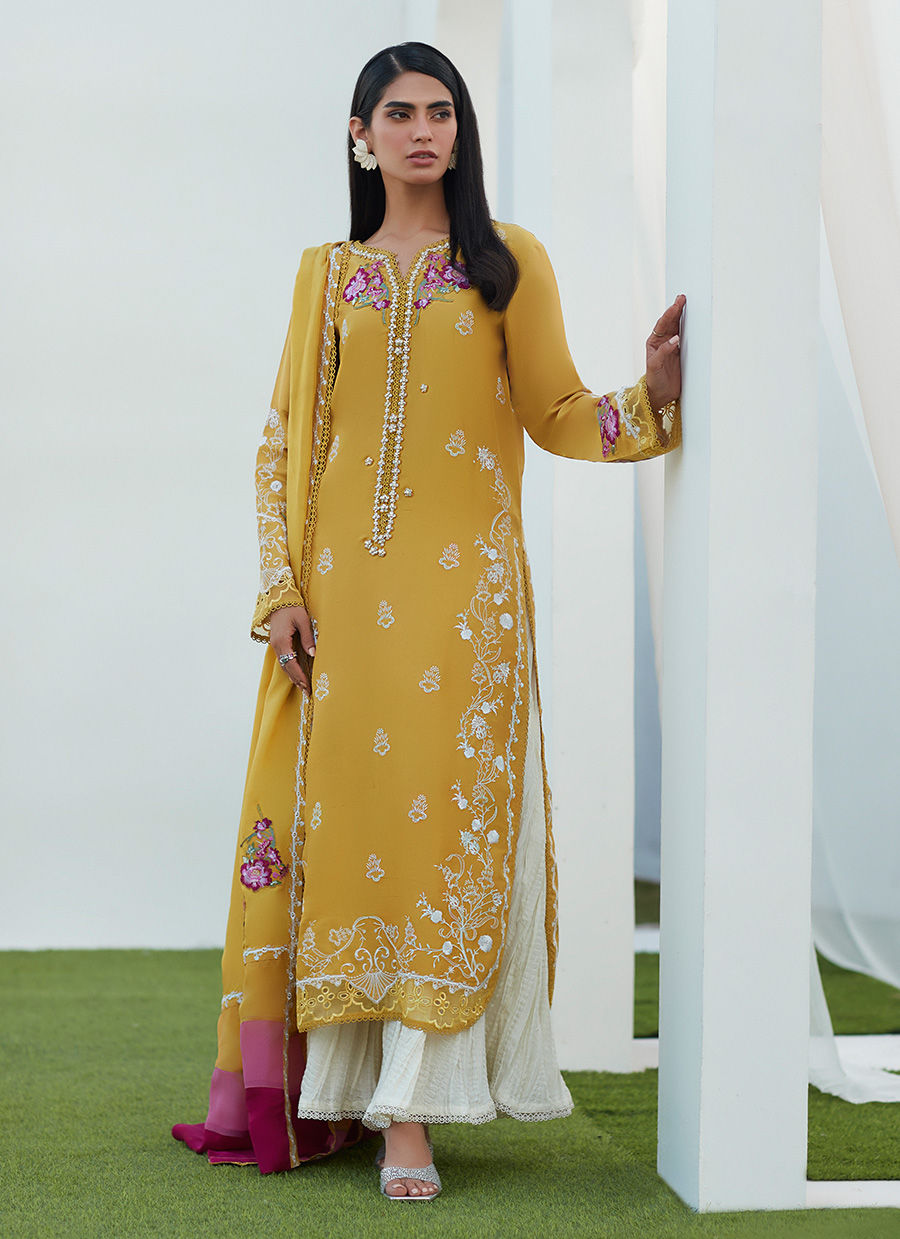This image portrays a young, attractive Indian woman with long black hair, standing gracefully on a green astroturf floor inside a white tent-like structure adorned with flowy curtains. She is dressed in a stunning, traditional mustard-colored (dark yellow) long-sleeve outfit, possibly a sari or dress, with intricate embroidery and beadwork in hues of pink, red, and green adorning the front, hem, and the wrists. The embroidery features a mix of floral patterns and filigree designs, with beadwork around the collar resembling small pearls or stars. She has a shawl or dupatta attached to one shoulder that drapes elegantly down to her feet, bordered with different shades of pink and maroon trim. The woman accessorizes with striking white earrings that resemble fanned-out petals or seashells. She is positioned with her hand resting on a white column or wooden support beam, looking off to the right, exuding the poise and grace of a model. The setting is enhanced by the white fabric draped around the columns, adding to the ethereal ambiance created by the ambient light filtering through.